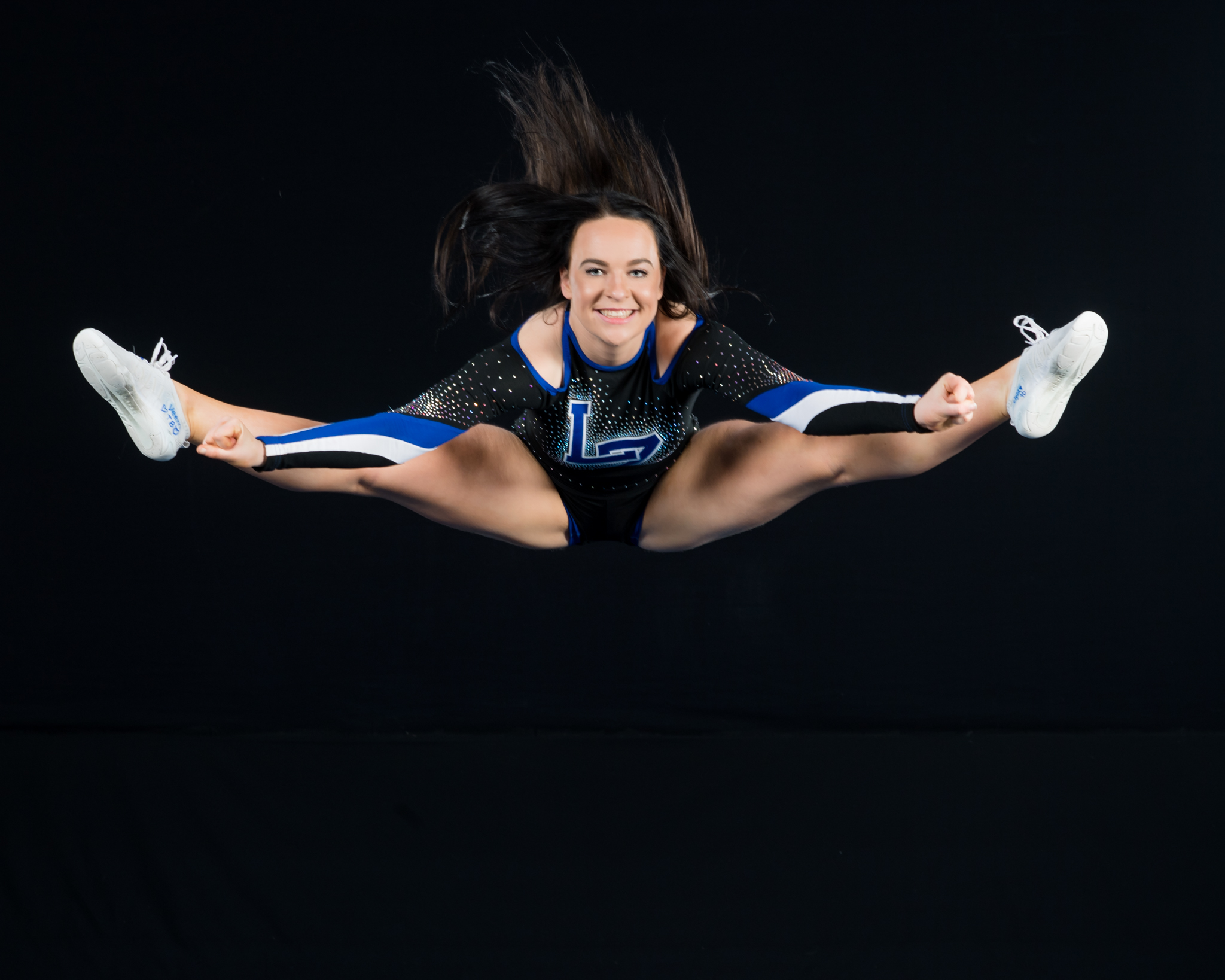In this captivating photograph, a smiling female cheerleader is captured mid-jump against a stark black background, emphasizing her athletic prowess and vibrant attire. She is suspended in the air, with her legs fully extended horizontally in a near-splits position from left to right, highlighting her flexibility and strength. Her arms are stretched out sideways, parallel to her legs, with her hands clenched into fists pointing towards her feet, creating a dynamic and symmetrical visual. She is dressed in a sequined, long-sleeve black bodysuit adorned with blue, white, and black stripes along the sleeves. The chest of her leotard features a prominently positioned blue letter 'L,' intersected by another partially obscured letter. Her long black hair flows upward dramatically, a testament to the velocity and energy of her leap. She completes the look with pristine white sneakers, her bare legs accentuated by the dark background which isolates her movement and showcases her feat. The photo captures her centered near the top of the frame, making her the sole focus of this impressive and electrifying image.